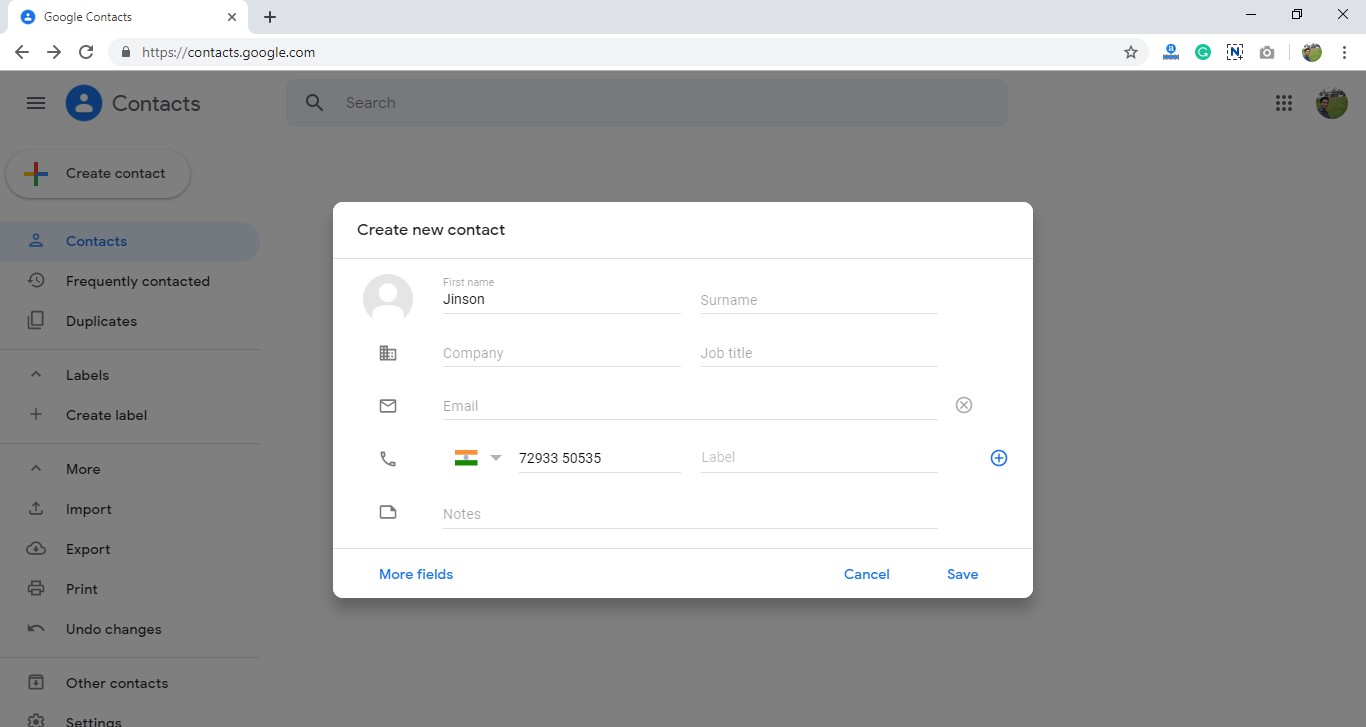The image depicts a screen capture in landscape mode with the Google Contacts interface open. The main content of the Google Contacts page is obscured by a dialog box in the foreground, which features a white background, graying out the underlying page including a vertical menu on the left side.

The dialog box is prominently titled "Create New Contact." Within this dialog box, there is a placeholder head-and-shoulders icon inside a circle, followed by several fields for contact information. The "First Name" field is filled with the name "Jinson," while the "Surname," "Company," "Job Title," and "Email" fields are empty. Below these form fields, there's a phone icon accompanied by an Indian flag and a phone number, "729-335-0535."

Additionally, a "Label" entry box is present with a plus sign encased in a circle icon to its right, allowing for additional customization. Further down is a "Notes" section illustrated by a notepad icon. At the bottom of the dialog box, there are blue links labeled "More fields," and buttons labeled "Cancel" and "Save" for finalizing or discarding the contact entry.